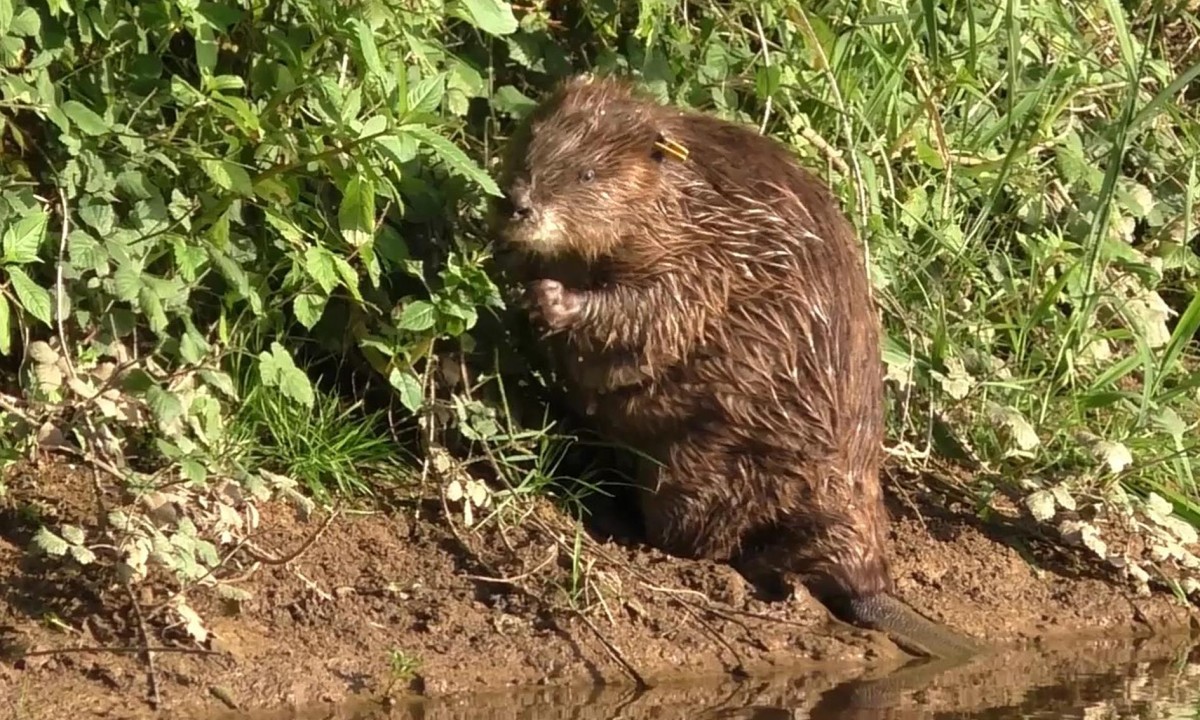In this bright daytime outdoor picture, a beaver is seen crouching over the muddy banks of a body of water. The beaver, which looks slightly scared with wide-open eyes, appears plump, suggesting it eats well. Its brown fur seems wet, likely from being in the water, and it has a notable yellow tag attached to its left ear. The beaver has its arms up towards its mouth, possibly clasping something it is chewing on. Surrounding the beaver, the ground is littered with twigs, branches, and dried, crumpled leaves. In the background, vibrant green grass and shrubs add a lush contrast to the muddy setting. The reflective muddy water further emphasizes the beaver's damp surroundings.